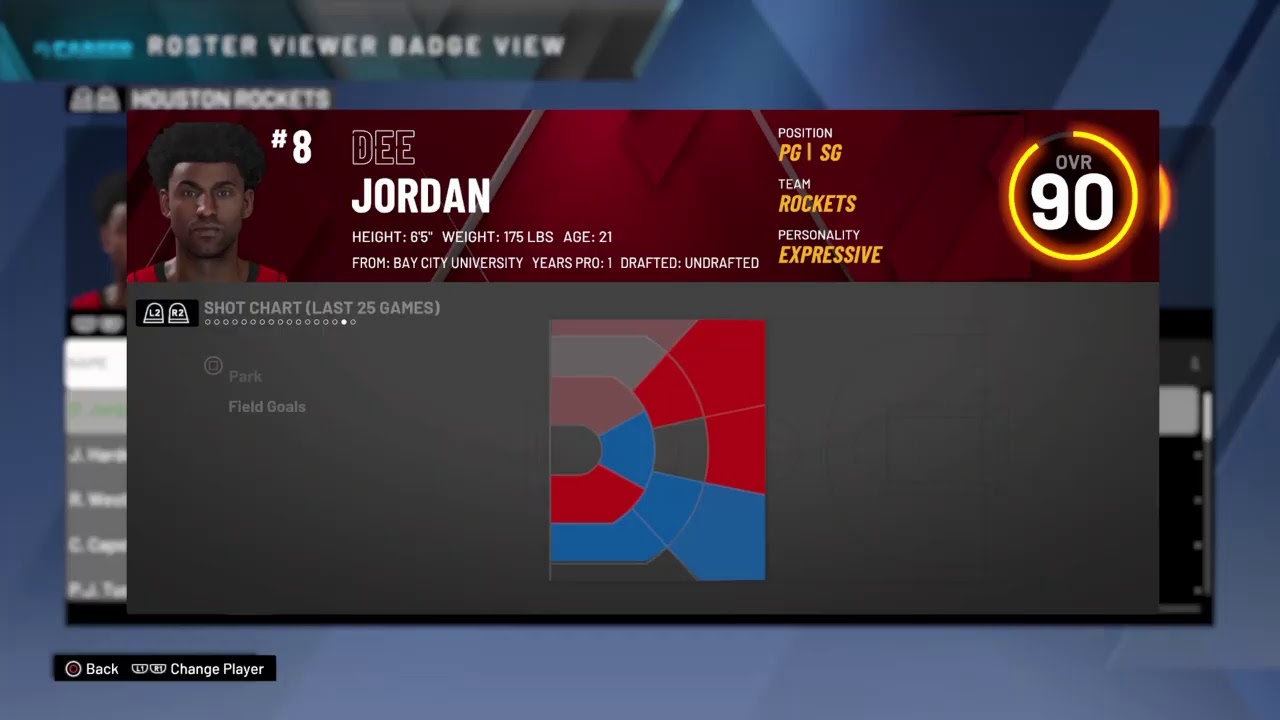The image is a highly detailed, panoramic sports statistics screen, predominantly featuring a profile of an African American male football player donning a red jersey with the number 8. The central focus is a long, clear rectangular section that highlights the player's stats. Above this section, a vibrant orange bar showcases the player's information, including his name, Jordan, displayed in distinct white letters, and his physical stats: height 6'5", weight 175 lbs, and age 21. 

Beneath this, "Bay City University" is specified along with career notes, "Pro 1" and "drafted: undrafted." Adjacent to the player's information, in the top right, are details of his playing positions indicated by "PG" (point guard) and "SG" (shooting guard), both in orange letters. The team name, "Rockets," is prominently shown in a combination of red and orange text, along with a label "expressive" in all caps orange.

To the far right, a bright orange circle is visible, nearly complete except for a small gray segment, containing the text "OVR 90" signifying the player's overall rating. Below the circle is a gray box featuring a multicolored, intricate design, possibly a logo or a seating chart, predominantly in shades of red, blue, and gray.

On the upper left, there's a black box with faint white symbols, the function of which is unclear. Directly to the right, the text reads "shot chart (last 25 games)" in pale white, capital letters. Below this are several gray-bordered circles arranged in a sequence, with the penultimate one filled in white. Further down, there is a faint gray circle with a square emblem and the word "park" nearby, followed by "field goal" in slightly brighter gray text.

The background shows a blurred blue area with partial images of the player and additional unreadable stats, enclosed by a blue boundary. At the very top of the image, the blurred text is in aqua blue alongside clearly visible large white capitalized words: "ROSTER," "VIEWER," "BADGE VIEW," and "HOUSTON ROCKETS." Two padlocks are faintly visible behind black backgrounds, indicating secured options.

In the lower left section, a long black box contains the white word "back," with a white-rimmed circle having an indistinct red interior to its left. Further right, two half circles with illegible contents precede the white letters "change player." Overall, the image appears to be a comprehensive sports statistics interface, likely for a football player from the Houston Rockets, detailing extensive personal and career information.